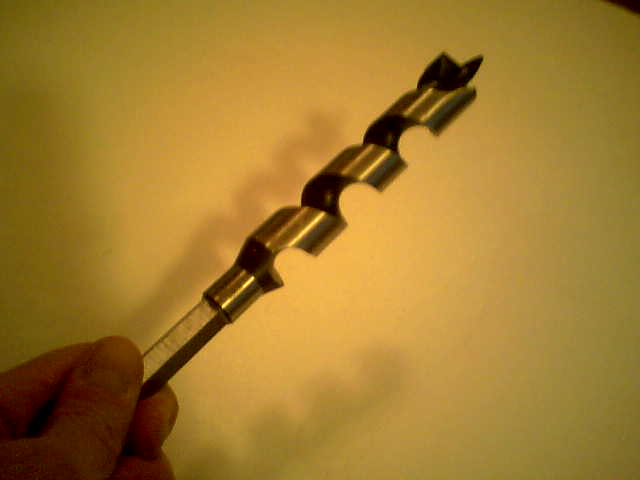The image features a hand grasping a spiral drill bit against a plain white background, likely a piece of paper. The fingers and thumb are partially visible, securing the drill bit, which appears to be approximately four to five inches in length. The drill bit, designed for penetrating walls, casts a shadow onto the background, adding dimensionality to the scene. The photograph is poorly lit, resulting in a murky yellowish tone, suggesting no flash photography was employed. Overall, the image is simple and devoid of context, primarily highlighting the hand and the drill bit.